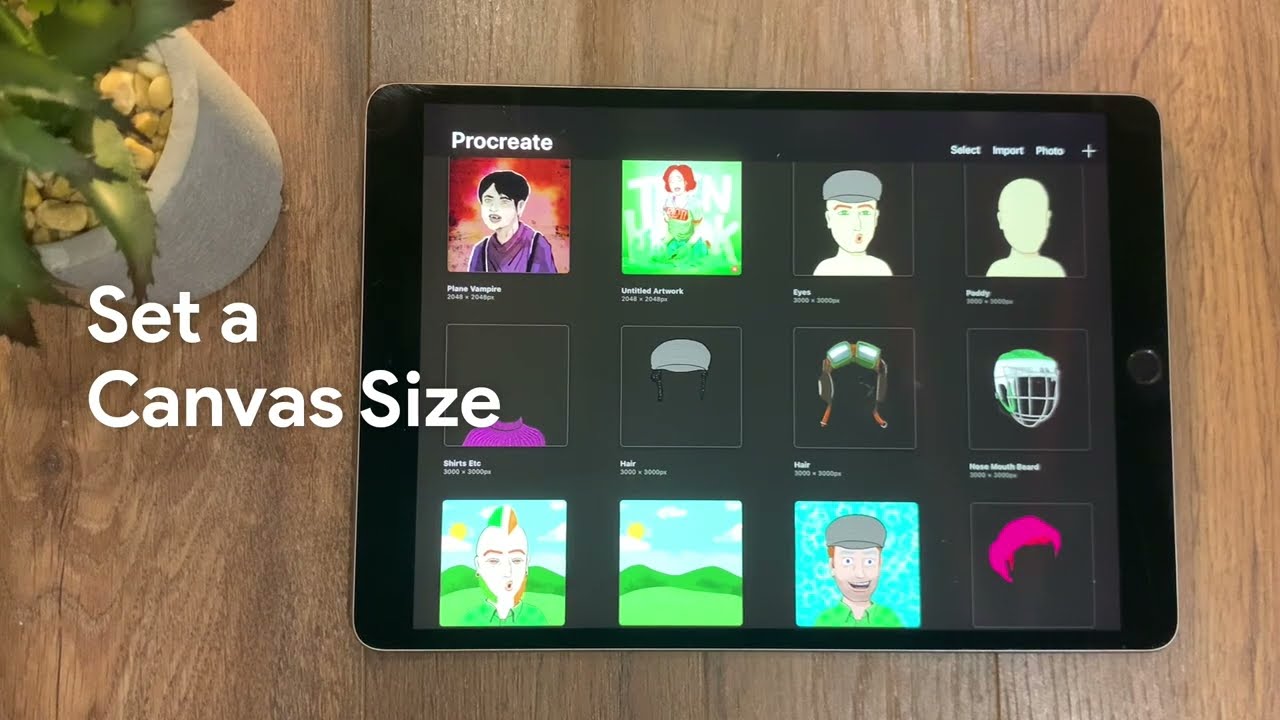This image features a black tablet lying on a brown wooden table, the wood grain running vertically. In the top left corner of the table, there's a small gray planter with yellow pebbles and green leaves. The photograph is taken from above, giving a clear view of the tablet's screen. The tablet, in landscape orientation, displays a grid of 12 thumbnail images, organized in four columns and three rows. These thumbnails depict cartoon heads of people and various headgear, including a silhouette of a head, aviation goggles, and a hockey helmet. In the upper left corner of the screen, the word "Procreate" is written in white letters. Additional white text options "Select" and "Import Photo" appear in the top right, along with a plus sign. On the left side of the screen, the phrase "Set a Canvas Size" is prominently displayed in white lettering.